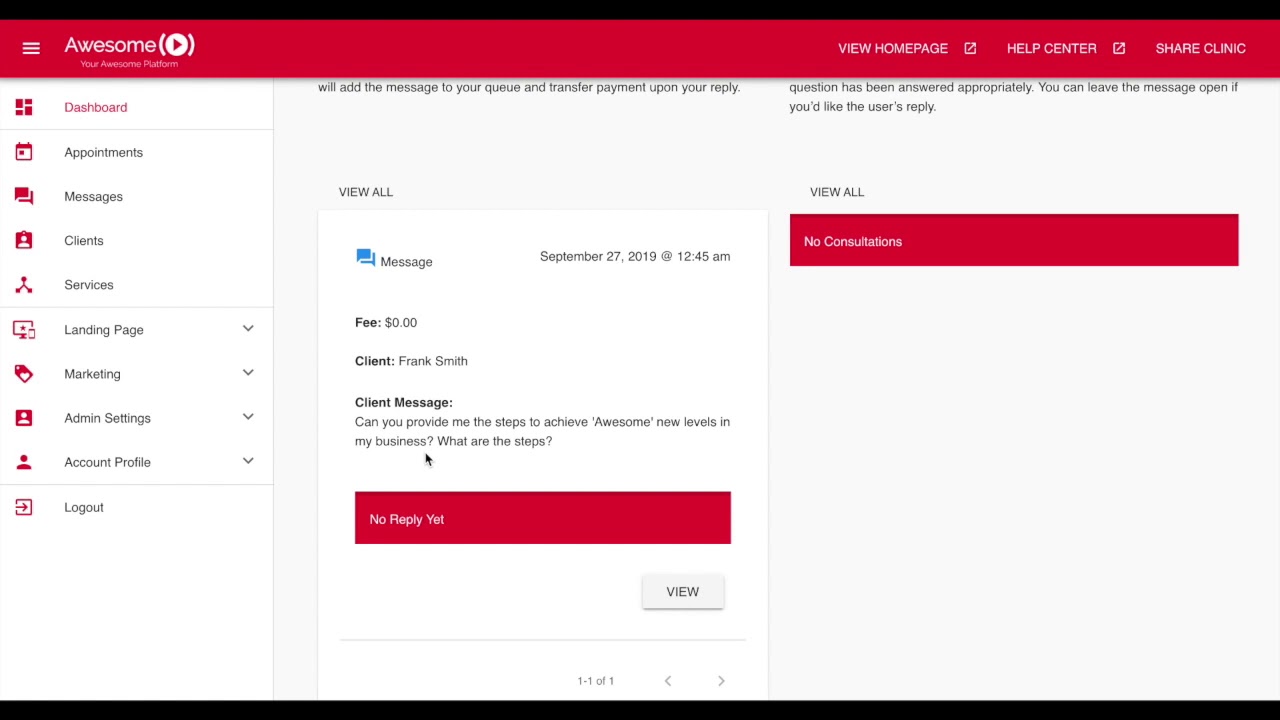This image, sourced from a website labeled "awesome," features various interface elements and text details. At the top of the image, there is a multicolored bar, split into black and red sections, with white text. In the upper left corner on the red portion of the bar, there's a white "list" button. Centrally located on the red bar is the word "awesome" in white text, accompanied by a white "play" button to its right. Further to the right on this bar, the text reads: "View Home Page | Help Center | Shape | Share | Clinic".

Running down the left side of the image, there is a vertical menu with the following items listed: Dashboard, Messages, Services, Clients, Landing Page, Marketing, Account, Profile, Admin Settings, and Log Out.

In the center of the image, there is a pop-up message related to a fee, providing important information to the user. On the right side of the image, there's a "View All" button, and below it, the text indicates "No consultants" or "No consultations" are available at the moment. The interface elements and textual components suggest this is likely a screenshot of a web application's dashboard or user interface.